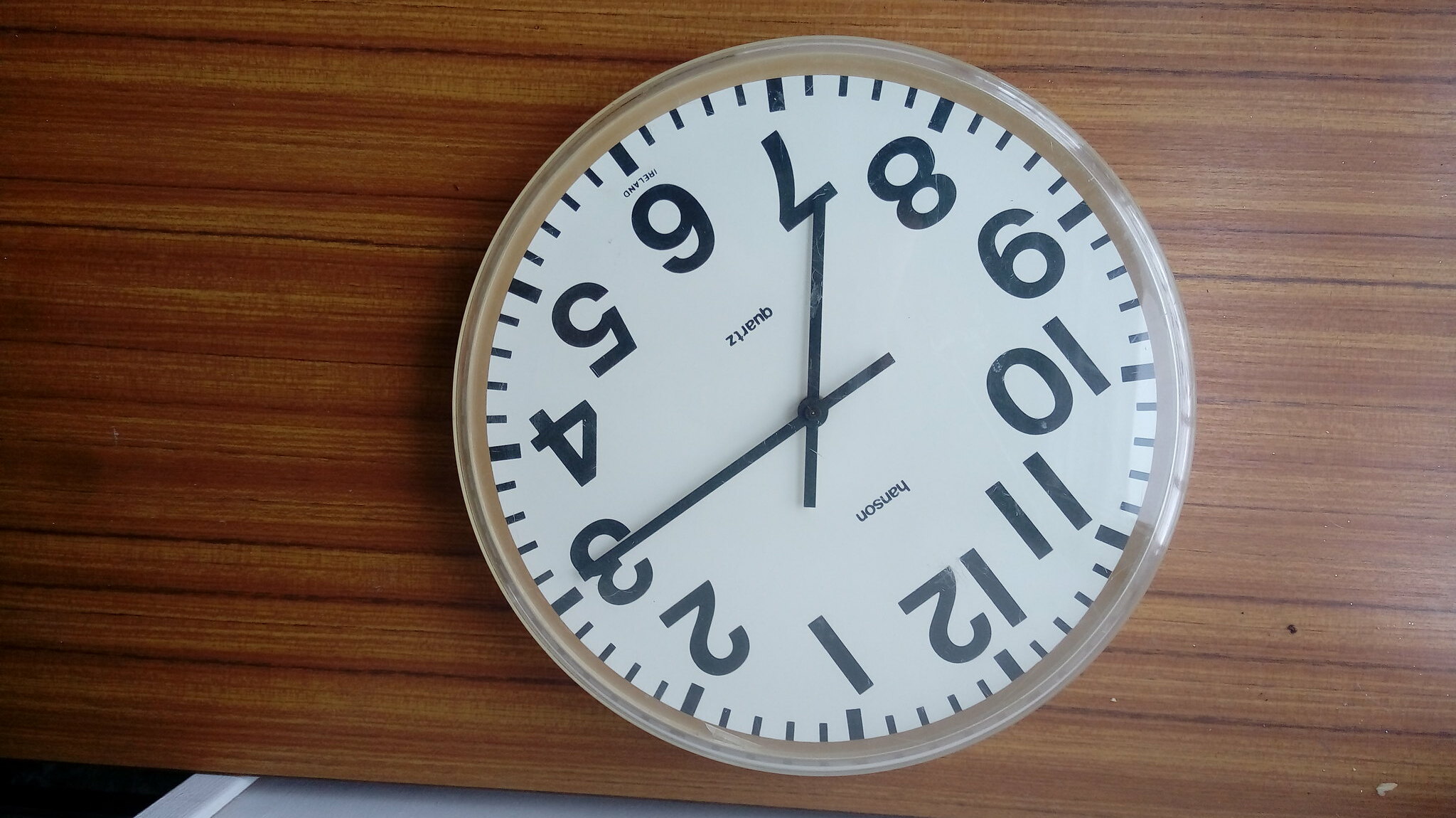This color photograph captures an analog wall clock placed peculiarly on a piece of grained wood, which appears to be a maple-toned, medium to dark brown surface. The clock is notably upside down and rotated at an angle. The clock face is white with clearly visible black numbers and small dashes marking the minutes. The numeral 7 is at the top, and the numeral 1 is at the bottom, giving the impression that the 12 is in the bottom left-hand corner. The clock shows the time as 7:15, with the shorter hour hand pointing towards the 7 and the longer minute hand pointing towards the 3. Surrounding the clock face is a light tan or chrome-like frame that is slightly reflective, indicating it might be older. The label "Quartz" is printed just above the 6, while the brand name "Hansen" appears below the 12. This clock, tilted and requiring head adjustment to view upright, rests on the wood surface, with a small white or cream-colored area visible on the surface's bottom left, possibly reflecting some light. The overall atmosphere of the image suggests a vintage quality, enhanced by the natural textures and tones of the wood and the clock's classic design.